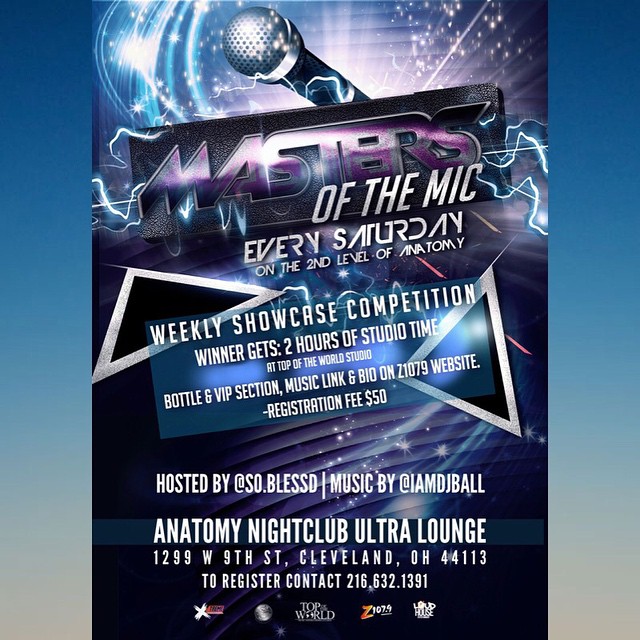The flyer is a detailed advertisement for a weekly music event titled "Masters of the Mic." The background on both sides features a gradient effect, transitioning from a darker blue at the top to a lighter blue and eventually gray at the bottom. The top section of the poster showcases starbursts and light effects, accentuating a prominently displayed 3D rendered microphone angled towards the top left corner.

Central to the flyer is the event's logo, a black square with "Masters" written in large purple text, overlaid by the microphone graphic. Below this, in white text, the flyer announces: "Every Saturday on the Second Level of Anatomy." A semi-transparent blue rectangle contains additional white text reading: "Weekly Showcase Competition." The subtext highlights the event's key detail: "Winner Gets 2 Hours of Studio Time at Top of the World Studio."

Further details include the registration fee of $50 and information about the event's location: "Anatomy Nightclub Ultra Lounge, 1299 West 9th Street, Cleveland, Ohio 44113." The poster also mentions the host and references a bottle and VIP section, with music linked on the Z1079 website. At the bottom are several station logos, adding to the flyer’s professional appeal.